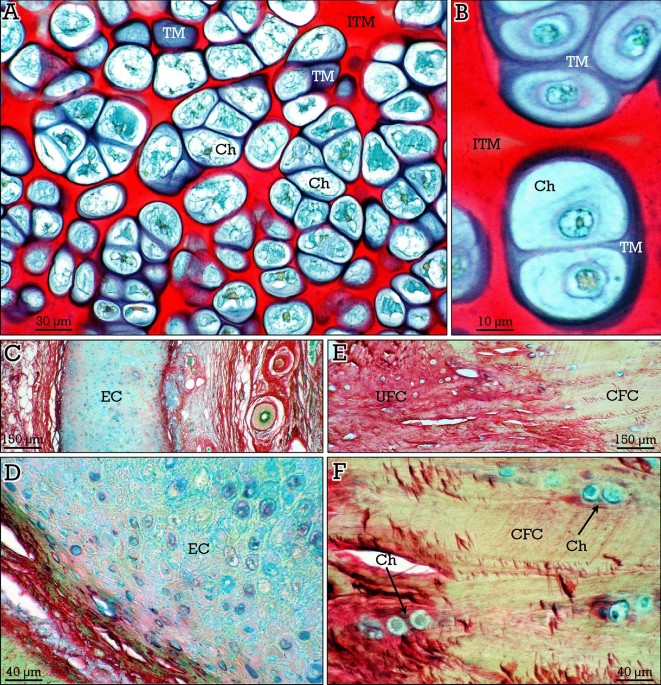The image is a detailed scientific diagram showcasing various up-close views of cellular or microbial structures under a microscope, arranged in a grid of six images (two rows of three). The top left image, labeled 'A,' depicts cells with light blue structures set against a vivid red gradient background. Various acronyms such as T-M, I-T-M, and C-H are marked around the cells, which appear to be bunched together. 'B,' the top right image, zooms in further, revealing intricate details of the cell structures. At the bottom left, text indicates a scale of 30 micrometers, emphasizing the microscopic scale. Images in the second row continue this close examination, with the fourth and fifth images providing even closer views at a scale of 40 micrometers, highlighting finer cell details and internal structures. The cells in these images vary in color, including shades of blue, greenish-blue, and reddish-orange. Each image is marked with scientific abbreviations, drawing attention to specific features within the cells.